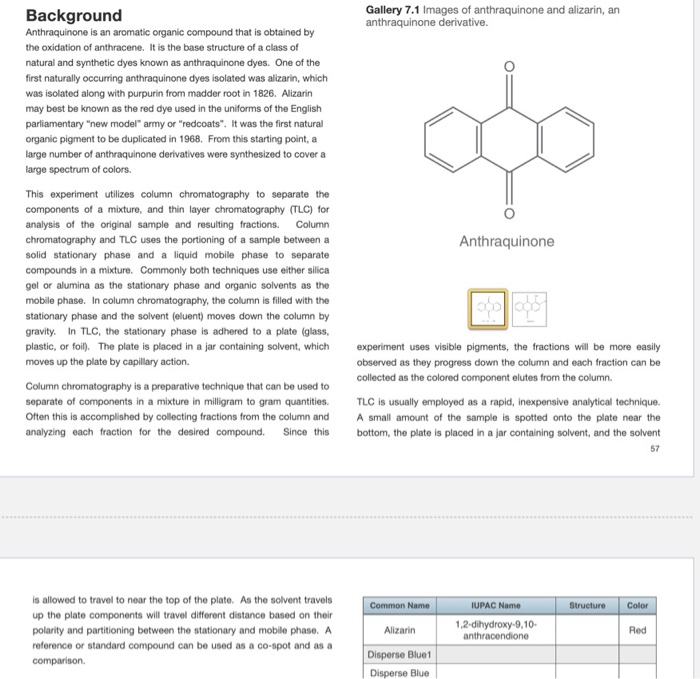This image, likely taken from a textbook or similar educational resource, illustrates the chemical structure and properties of anthraquinone, an aromatic organic compound obtained through the oxidation of anthracene. The structure, shown in detail, features three joined hexagonal shapes with two bars extending from the center top and bottom, ending in circles. This page, titled "Gallery 7.1," includes images of anthraquinone, alizarin, and various anthraquinone derivatives. The page is divided into two columns; the left column provides a detailed description, starting with the chemical background of anthraquinone and highlighting its significance in natural and synthetic dyes, including the historical isolation of alizarin in 1826. The right column includes a visual representation of anthraquinone's hexagonal structure and a table at the bottom listing chemical names, IUPAC names, structures, and colors of related compounds like alizarin and disperse blue. The complexity of the information and terminology suggests it is intended as a learning tool for science students.